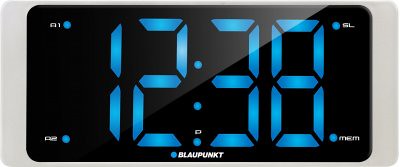The image features a digital clock with a sleek, rectangular design. The clock's black screen vividly showcases the time "12:38" in bright blue LED numerals. Each numeral is crisply outlined, offering a clear and modern look. Below the numbers, there's a small blue dot and the brand name "BLAUPUNKT" displayed prominently in white, all caps lettering. 

In the four corners of the screen, small blue dots are present with additional textual markings. The top left corner is marked "A1" and the bottom left reads "A2." The top right corner features another blue dot followed by the letters "SL." The bottom right corner also has a blue dot, with the letters "MEM" beside it, likely indicating a memory function.

Between the hour and minute digits, two standard blue dots are visible, typical of digital clocks. Additionally, a third blue dot appears below these central dots, and above them sits an enigmatic small white circle, adding a unique element to the clock's design.